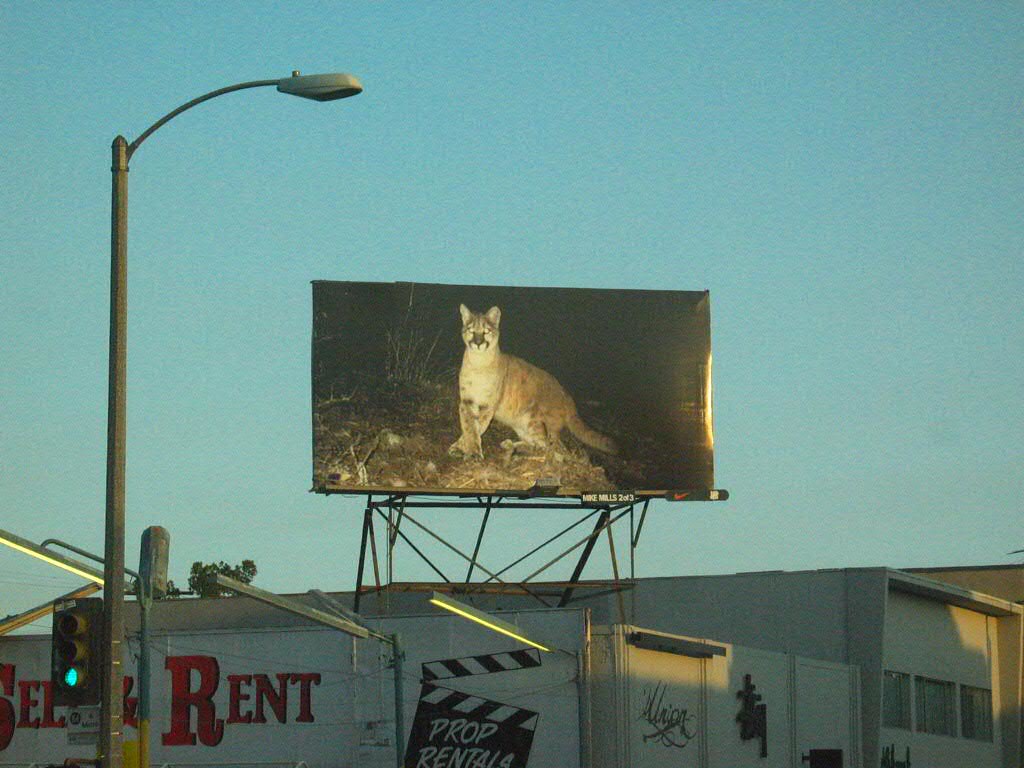A rectangular white building features a large billboard on its rooftop that prominently displays the word "RENT" in bold, red letters. Below the text, the billboard showcases an illustration of a classic director's slate—a black square with a hinged top adorned with white and black stripes, traditionally used to mark the beginning of filming scenes. The slate graphic includes the text "Prop Rentals" spelled out in white capital letters.

Adjacent to the right side of the building's facade is a patch of black graffiti, seemingly created with spray paint. On the left side of the building, a street light stands next to a traffic light, which is currently showing a green signal. Mounted on the rooftop billboard, there's also an image of a bobcat, depicted as a large, brown feline gazing out over the city.